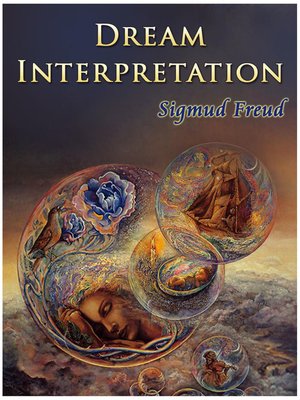The cover image of the book "Dream Interpretation" by Sigmund Freud features a striking, dark blue background with clouds resembling a high-altitude sky. At the top, the title "Dream Interpretation" is prominently displayed in large yellow text, while just below, the author’s name, Sigmund Freud, is written in blue letters. The centerpiece of the cover is an artistic depiction of multiple floating orbs filled with vivid, dreamlike imagery. The largest orb, situated to the middle left, contains the serene face of a woman lying on her right side, her eyes and mouth closed, surrounded by swirls of yellow, pink, purple, and green hues. Above her, within the same orb, there's a delicate bird and two blue flowers outlined in pink. To the right of this central orb, two smaller bubbles are visible; one contains a tan figure, while the other, positioned slightly lower, showcases an oval cradle with a baby draped in a sash. Beneath the central orb, in the right corner, another bubble presents a person playing a violin. Scattered across the cover, additional orbs continue the dream motif, housing images like a sailing ship and more enigmatic figures, all against the backdrop of a dark, mystic sky.